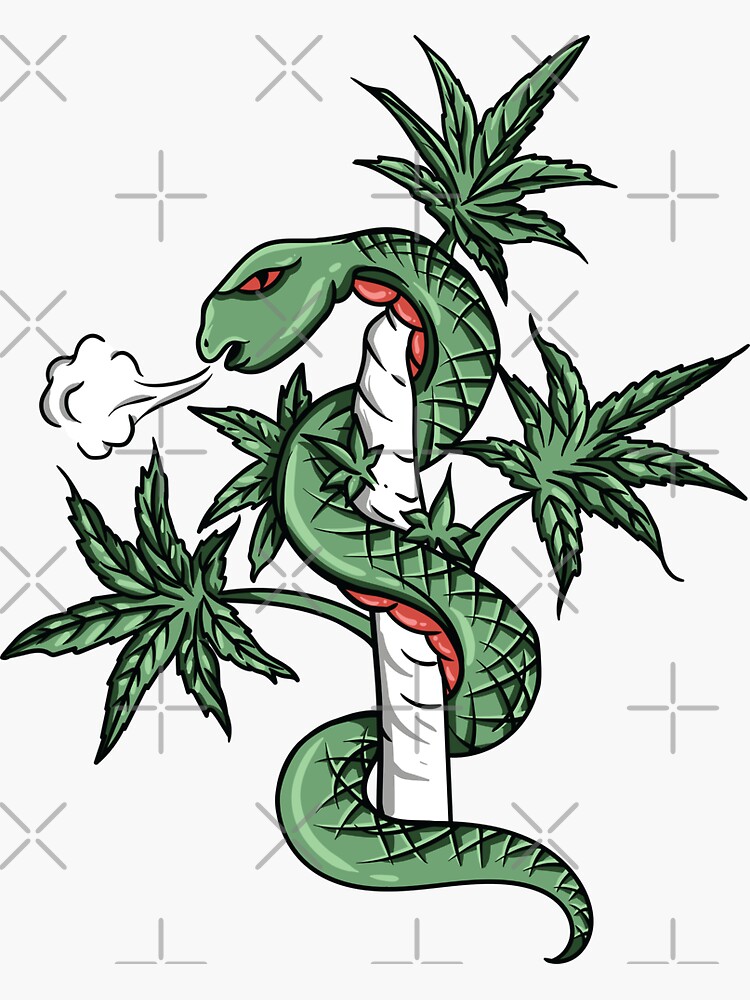This cartoon-like illustration features a vibrant green snake with a red eye encircling a white, twisted cylinder meant to depict a joint. The snake's body, accented with cross-hatched scales and a row of red scales along its stomach, undulates counterclockwise around the joint. Its open mouth emits a puff of white smoke. Surrounding the snake are several large, seven-leaved green marijuana leaves in various positions: one at the top, one below, one to the right, another just below the middle on the left, and two smaller ones in the center. The background is primarily white with a pattern of non-connecting gray pluses and Xs, which create blank spots at their intersections.